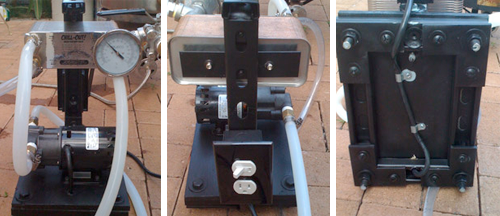The image is a three-panel, horizontally aligned photograph displaying different views of a complex measuring device, likely pneumatic or hydraulic. In the left panel, the front view is shown, featuring a silver rectangular box with a prominent dial gauge on its right side, indicating measurement activity. Below this box, two white tubes extend and connect to a cylinder-shaped attachment, all mounted on a black platform resting on a beige tiled floor.

The central panel offers a rear perspective of the device, showcasing the same rectangular silver box at the top, connected via a crossbeam to an outlet at the bottom, equipped with dual plug sockets. 

The right panel depicts the underside of the machine, revealing the black platform and a visible electrical cable running across it. Additionally, screws and feet are noticeable, holding the structure together. This detailed setup suggests a sophisticated piece of equipment designed for precise measurement tasks.